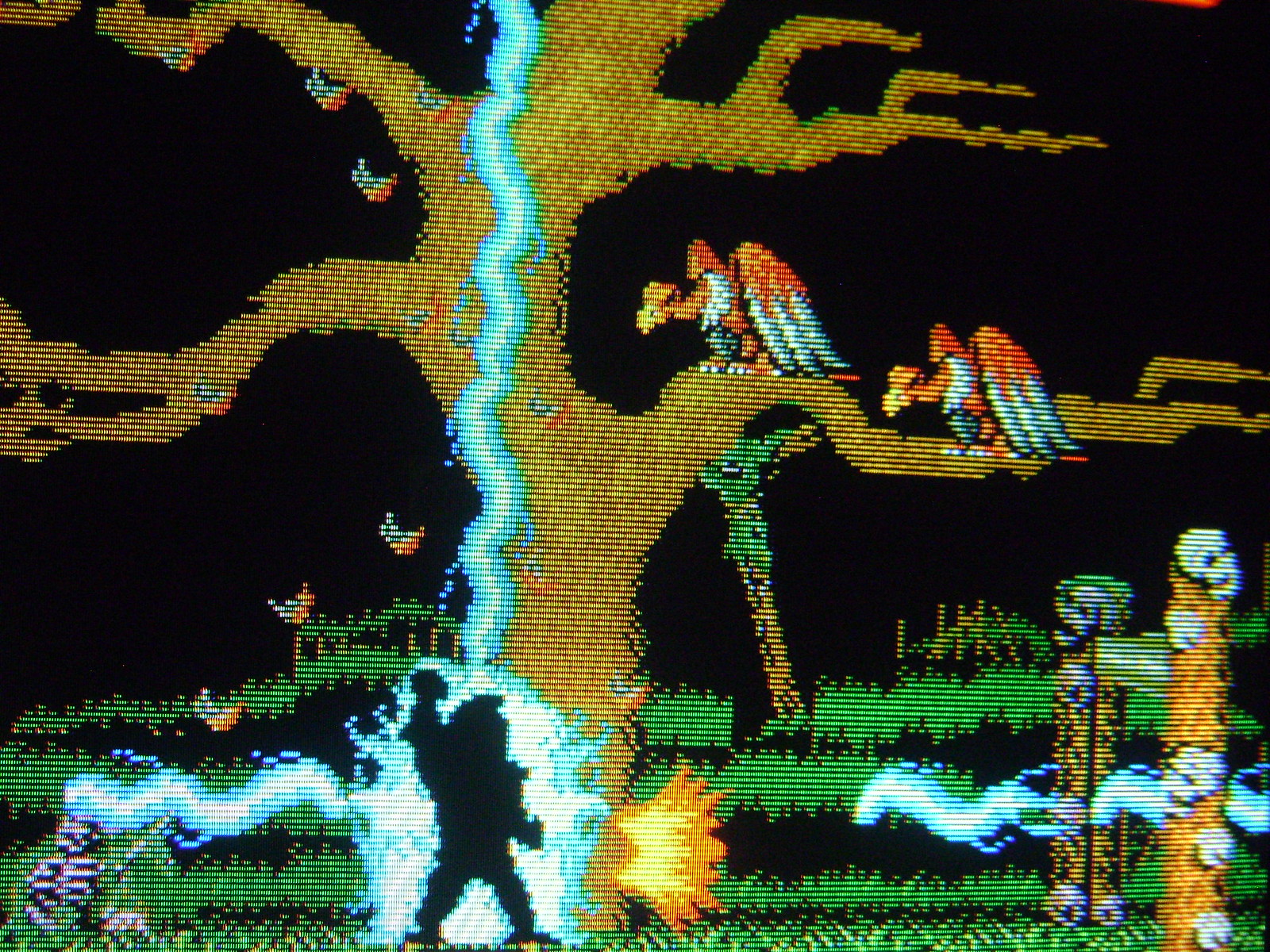This color image is a pixelated screenshot suggesting an old-fashioned video game from the Sega Genesis or Super Nintendo era, possibly earlier. Central to the scene is a large, leafless brown tree with four branches, two of which host hunched vultures with red and green wings and orange faces, appearing poised to pounce. To the right of the tree stands a brown ladder. At the base of the tree is a human-like figure illuminated by green light, raising its arm as green lightning bolts extend from it to the sides and above its head. The nighttime backdrop features a black sky, green grass, and scattered skulls—one perched on a yellow pole and another on a black and yellow spike. This tightly composed scene captures the eerie and detailed atmosphere of the game.